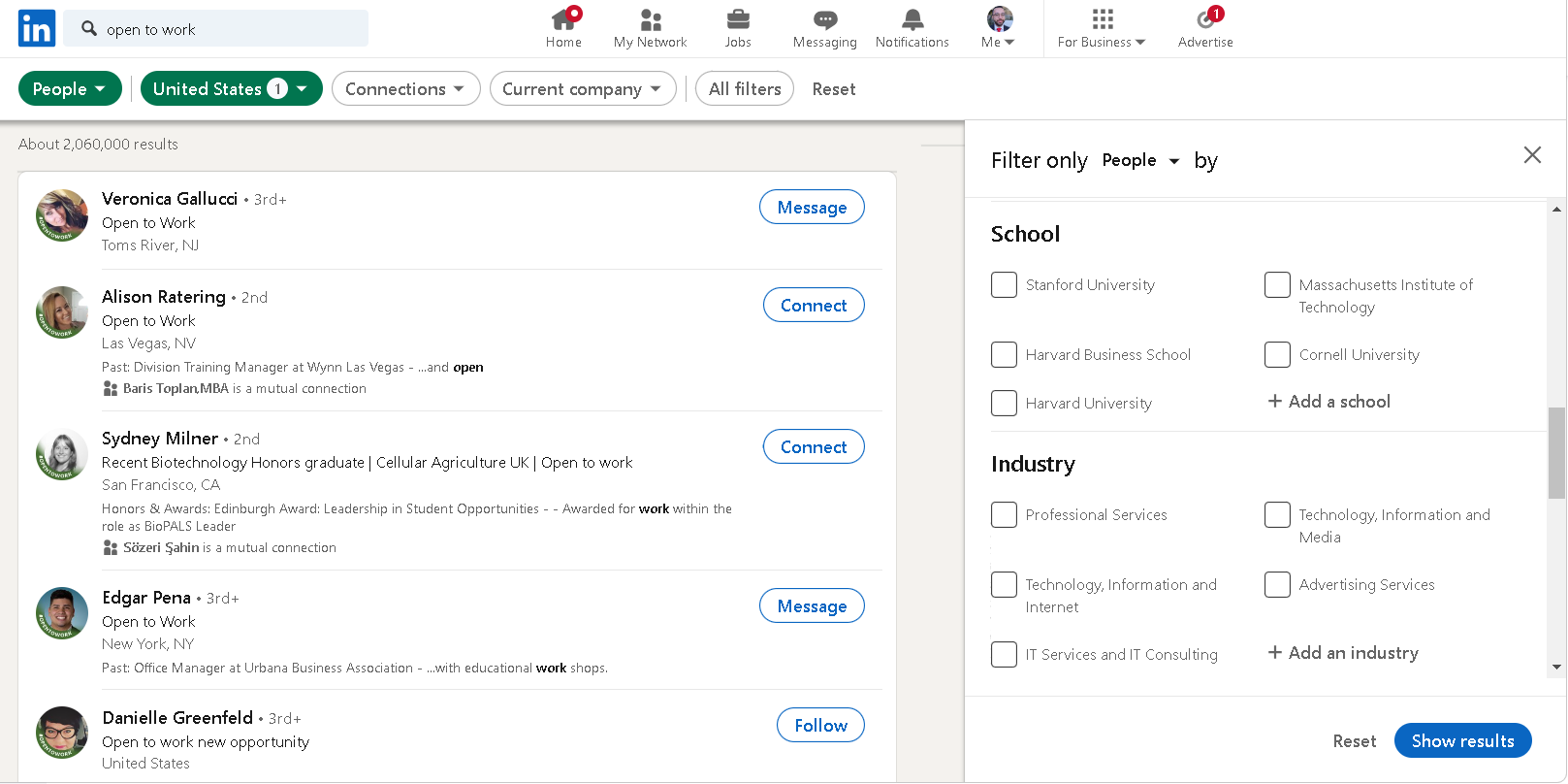This image is a detailed screenshot of the LinkedIn website interface. In the top left-hand corner, the recognizable LinkedIn logo is visible—a small blue square with the word "in" in white font. Along the left side of the screen, search results featuring various individuals are displayed. At the very top left, the search bar contains the text "Open to Work."

Five individual profiles are listed beneath the search bar, each showcasing the person's profile picture, name, location, and professional background. To the right of each profile, users have the options to message, connect, or follow the individual. These options are presented as white oval-shaped buttons with blue text.

On the right side of the screen, an open filter window titled "Filter Only People by School or Industry" is visible. At the bottom right, there is a blue "Show Results" button and a "Reset" button, used to refine the search. The website's background is primarily white, while the text appears in black, maintaining a clean and professional appearance.